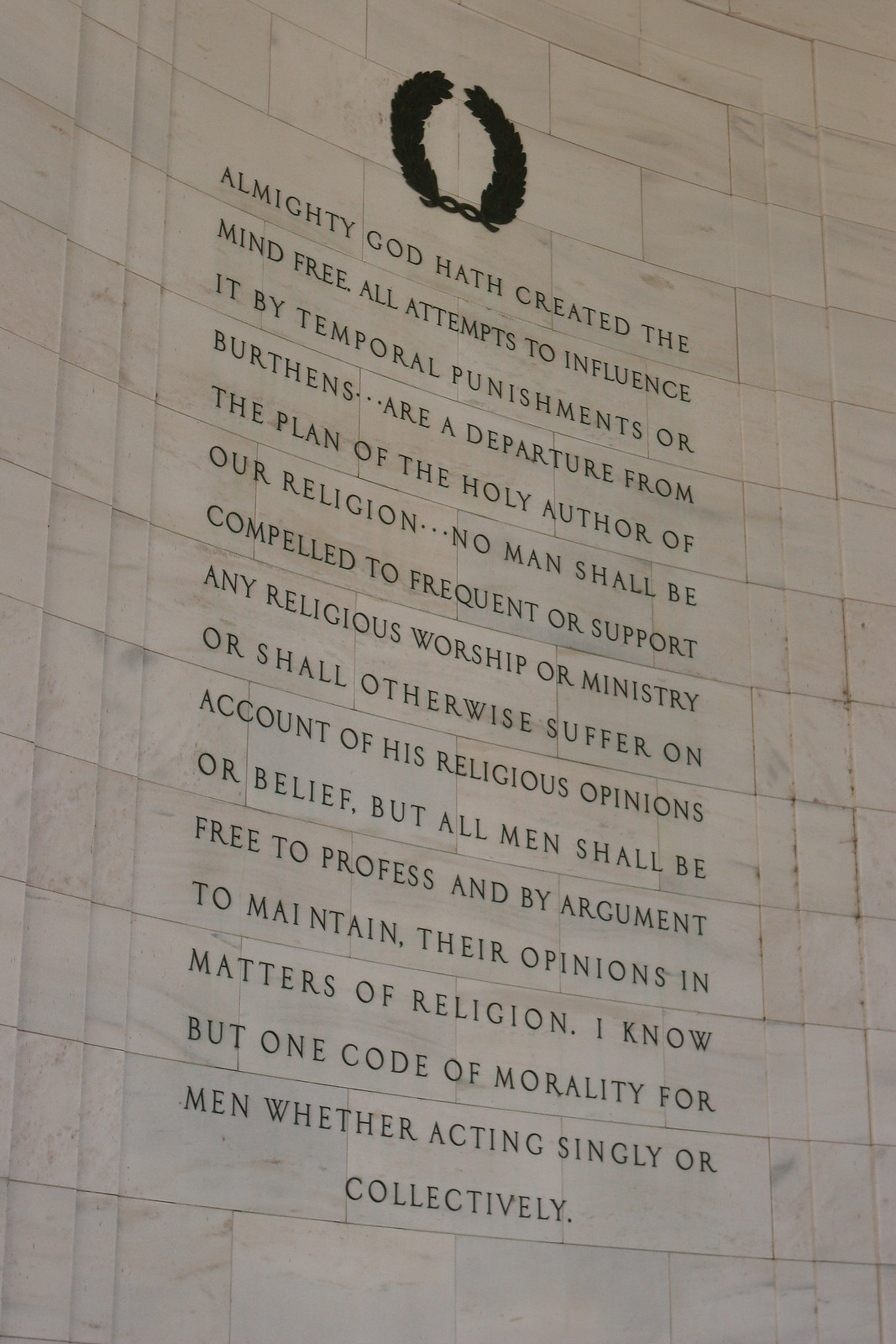The photograph captures a stately and majestic marble wall, cream-colored and composed of large interconnected slabs. At the top of the wall is a carved, double-sided open wreath in black, followed by a column of solemn black text. The inscription reads: "Almighty God hath created the mind free. All attempts to influence it by temporal punishment or burdens are a departure from the plan of the holy author of our religion. No man shall be compelled to frequent or support any religious worship or ministry, or shall otherwise suffer on account of his religious opinions or beliefs. But all men shall be free to profess and by argument to maintain their opinions in matters of religion. I know but one code of morality for men whether acting singly or collectively." The setting, detail, and evocative inscription suggest that this wall is part of a memorial structure, embodying a profound reverence for freedom and morality.